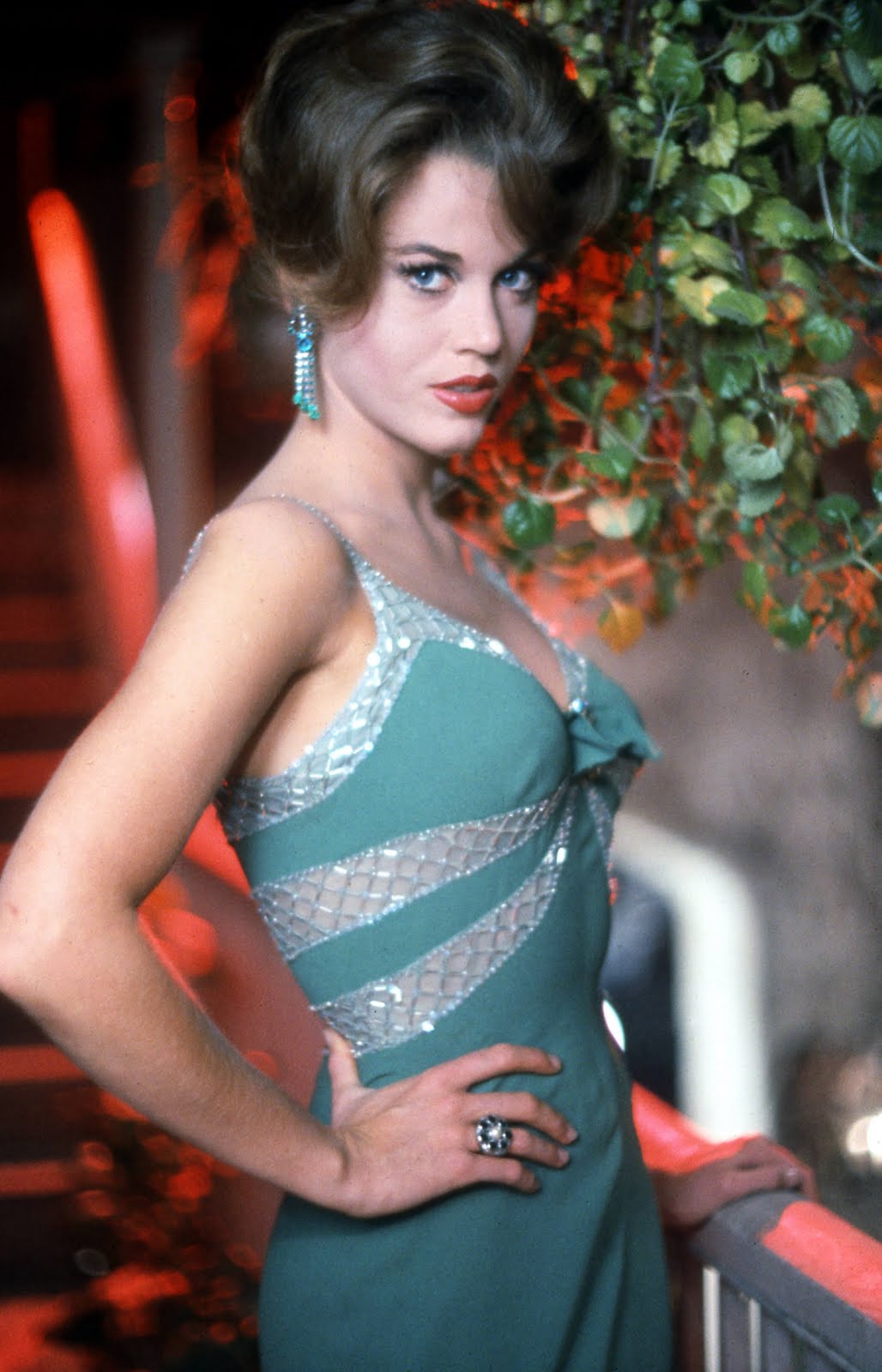The image presents a close-up of an elegant woman who appears to be a model or actress, embodying an old-school glamor. Her brown hair is styled in a sophisticated updo with wavy details in the front, perfectly placed to accentuate her features. She has striking blue eyes and is wearing bold red lipstick. Dangling from her ears are long, emerald green earrings that shimmer with intricate silver patterns.

Her attire is a stunning, long emerald green evening dress, adorned with exquisite silver beading and patterns predominantly concentrated at the upper part. The dress features thin straps and is gathered in the center, creating a bow-like effect that adds a touch of intricate elegance. She accessorizes with a ring adorning the ring finger of her right hand.

The background suggests an evening setting with a staircase lit up in red on the left side, creating dramatic splashes of red light behind her. To the top right of the image, green leaves hang down, adding a natural touch to the scene. Her pose is poised and graceful, with one hand placed on her hip and the other delicately touching a railing, as she gazes slightly upward while directly engaging with the camera.